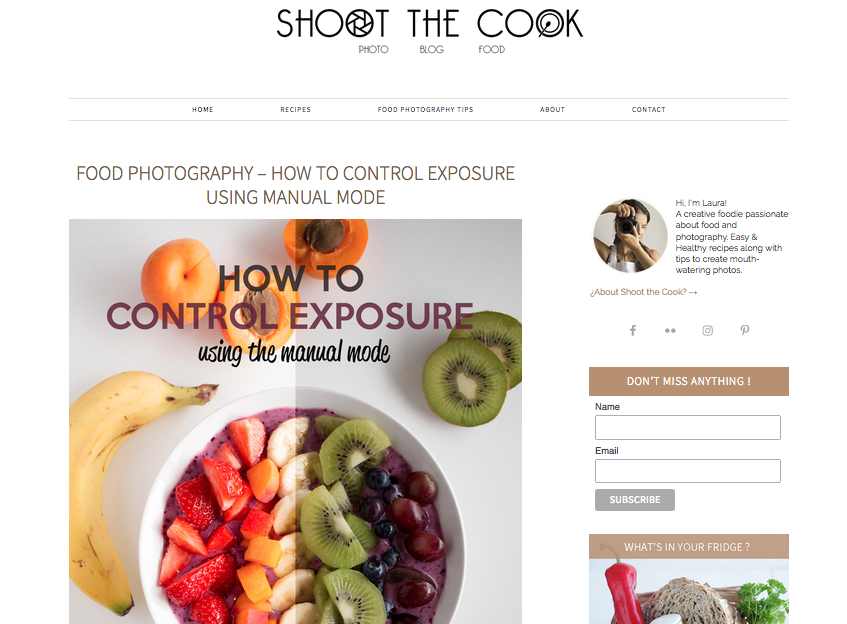At the top of the image, in bold black capital letters, it reads "SHOOT THE COOK." Below this, there is a tagline, "Photo Blog of Food," with a single horizontal line beneath it. Following that, there are two horizontal lines with a navigation menu in between, which includes sections labeled "Home," "Recipes," "Food Photography Tips," "About," and "Contact."

Below this navigation bar, the title reads "FOOD PHOTOGRAPHY – HOW TO CONTROL EXPOSURE USING MANUAL MODE." The accompanying image features a vibrant purple background. In the foreground, a pristine white bowl is filled with an assortment of fresh fruits including strawberries, mango slices, banana slices, kiwi, blueberries, and red grapes. To the left of the bowl, a banana is placed, while a few apricots are positioned above it. To the right of the bowl, a couple of kiwis can be seen.

On the right side of the image, the text "HOW TO CONTROL EXPOSURE USING MANUAL MODE" is reiterated. Below this, there’s a prompt labelled "Don’t Miss Anything," with two empty fields for users to input their name and email address.